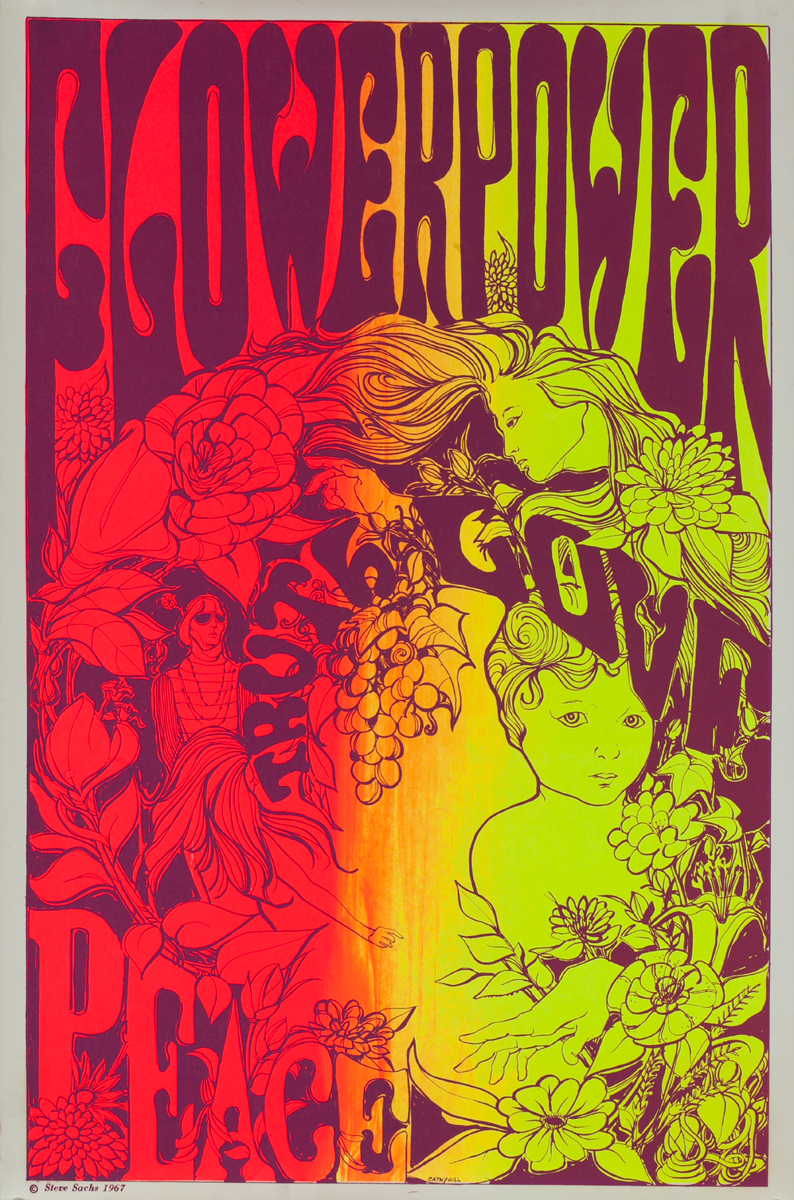The image is a colorful, psychedelic artwork resembling a poster, imbued with a trippy, surreal, and fantasy feel. Dominantly colored with vibrant reds on the left transitioning to oranges in the center, and yellowish-greens on the right, it has a striking color gradient. At the top, an arched text spell out "Flower Power" in a dark red-brown or dark purple ornate flower-shaped font. Below this, the scene unfolds with detailed imagery: 

On the right side, a woman with long, flowing hair that projects upward and to the left is adorned with flowers, which also emanate from her hair. To the left, another woman sits surrounded by fruits, and nearby vertically-curving text that transitions to a horizontal form reads "Truth" followed by what appears to be "Love" or something similar, although it's somewhat ambiguous. Lower in the image, there's a child or baby enveloped in flowers, and at the bottom left corner, the word "Peace" is prominently displayed. The overall theme suggests a blend of peace, love, and truth, reminiscent of a 1960s blacklight poster, suitable for a college dorm room or a tribute to a flower child era.